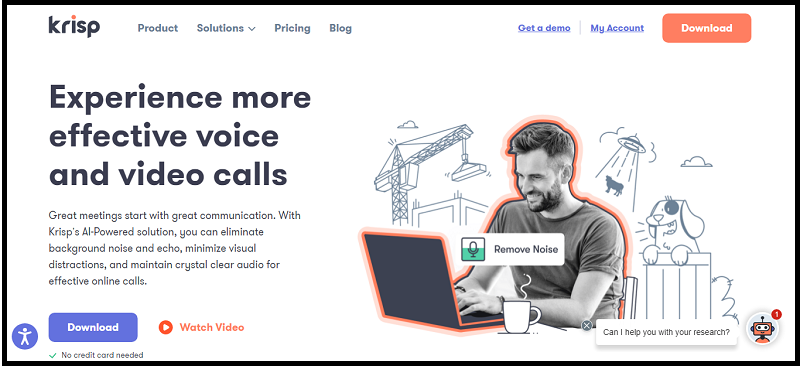A rectangular advertisement image, likely sourced from a website or app, promoting the company Crisp (spelled K-R-I-S-P), is displayed. The long side of the rectangle stretches from left to right. In the upper left-hand corner, "Crisp" is prominently featured in bold black text. Along the top, a navigation menu includes the options: "Product," "Solutions," "Pricing," and "Blog." Toward the right-hand side, links for "Get a demo" and "My account" are shown in blue and underlined, followed by an orange box with white text that reads "Download."

Below, a headline in large print states, "Experience more effective voice and video calls." A supporting sub-text in smaller font elaborates: "Great meetings start with great communication. With Crisp's AI-powered solution, you can eliminate background noise and echo, minimize visual distractions, and maintain crystal clear audio for effective online calls." Directly under this text, a blue button labeled "Download" and an orange link labeled "Watch video" are positioned.

On the right-hand side of the image, a person is depicted typing on a laptop, with illustrative images of noise sources in the background to suggest distractions that Crisp's technology can neutralize.